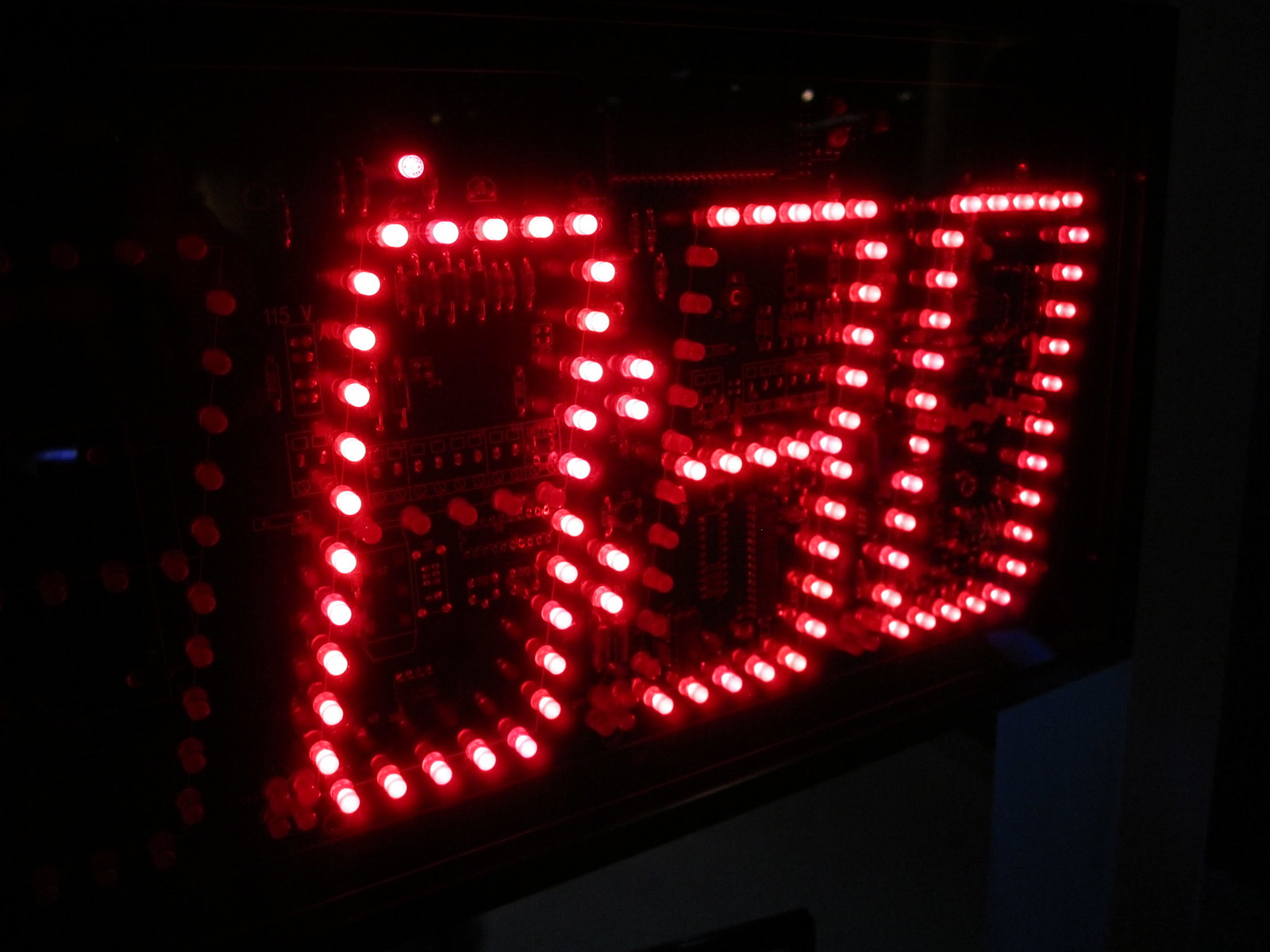The image features a close-up view of a digital clock display, prominently showing the numbers "030" composed of individual red glowing bulbs. Despite a predominantly black background, a faint blue horizontal line appears to the left center, adding subtle context to the otherwise minimalistic setting. The intricate design clearly reveals each tiny bulb forming the numbers, suggesting that the sign might be capable of changing its display. The bulbs’ illumination against the red backdrop highlights the detailed construction, possibly allowing observers to glimpse some of the clock's internal components. Notably, on the right side of the zero, there are markings resembling colons, hinting at the clock's typical time-keeping function.